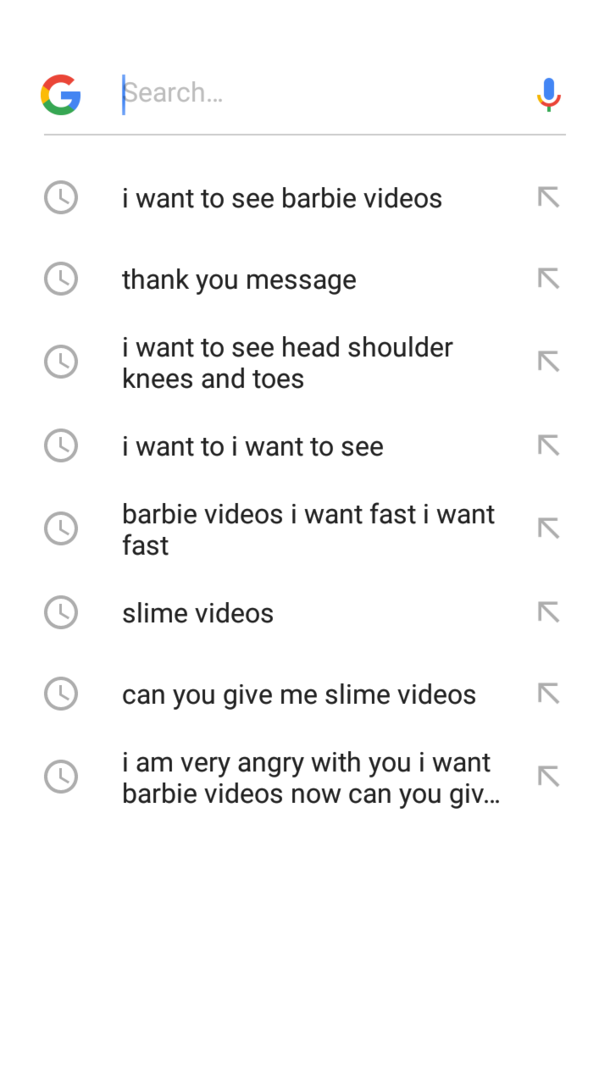In this image, a Google search interface is displayed prominently. At the top, there is the familiar Google search bar with the "Google Search" button clearly visible. The search bar features a faint blue line where users can type their inquiries, though it appears empty in this instance. 

To the right of the search bar, there is a small microphone icon indicating that users can also perform searches using voice commands.

Below the search bar, a series of recently conducted searches are listed, numbering eight in total. The first entry reads, "I want to see Barbie videos," followed by "thank you message." Subsequent entries include "I want to see head, shoulder, knees, and toes" and several repetitive searches starting with "I want to see." Further down, there are specific and somewhat frenzied searches like "Barbie videos, I want fast," "slime videos," and "can you give me slime videos?" The final search entry displays a more frustrated tone: "I am very angry with you, I want Barbie videos now, can you give?"

It appears that these search entries were made by a child, given their repetitive and emphatic nature, suggesting frustration over not being able to find the desired Barbie videos. 

The page itself has a clean and simple design with a white background, featuring the Google logo above the search box. On the left side of each search inquiry, there is a small clock icon, signifying a history log. On the right side of each search, there is an arrow pointing to the northwest.

Overall, the image gives a snapshot of a child’s attempts to find specific content on Google, resulting in a progressively exasperated series of search queries.